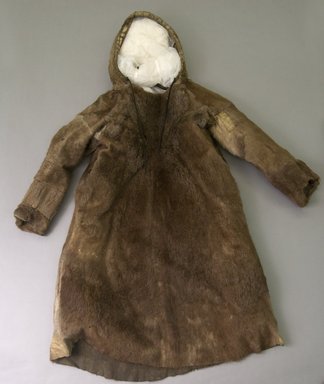The photograph showcases a vintage, worn hooded coat intended for a small child, possibly from the Aleutian Islands in Alaska or a northern Native American tribe. The coat is composed of brown fur skins with variegated patterns due to different pelts sewn together. It features long sleeves, slightly darker cuffs, and a hood that flares slightly from the chest down to the open bottom, creating a cone-like shape. The hood is propped open with white material, likely for photographic purposes, highlighting its design. The coat, with visible signs of wear, includes two long dark strings extending from the hood down the chest. The entire ensemble is captured against a gray background, emphasizing the brown, gray, and white color palette.